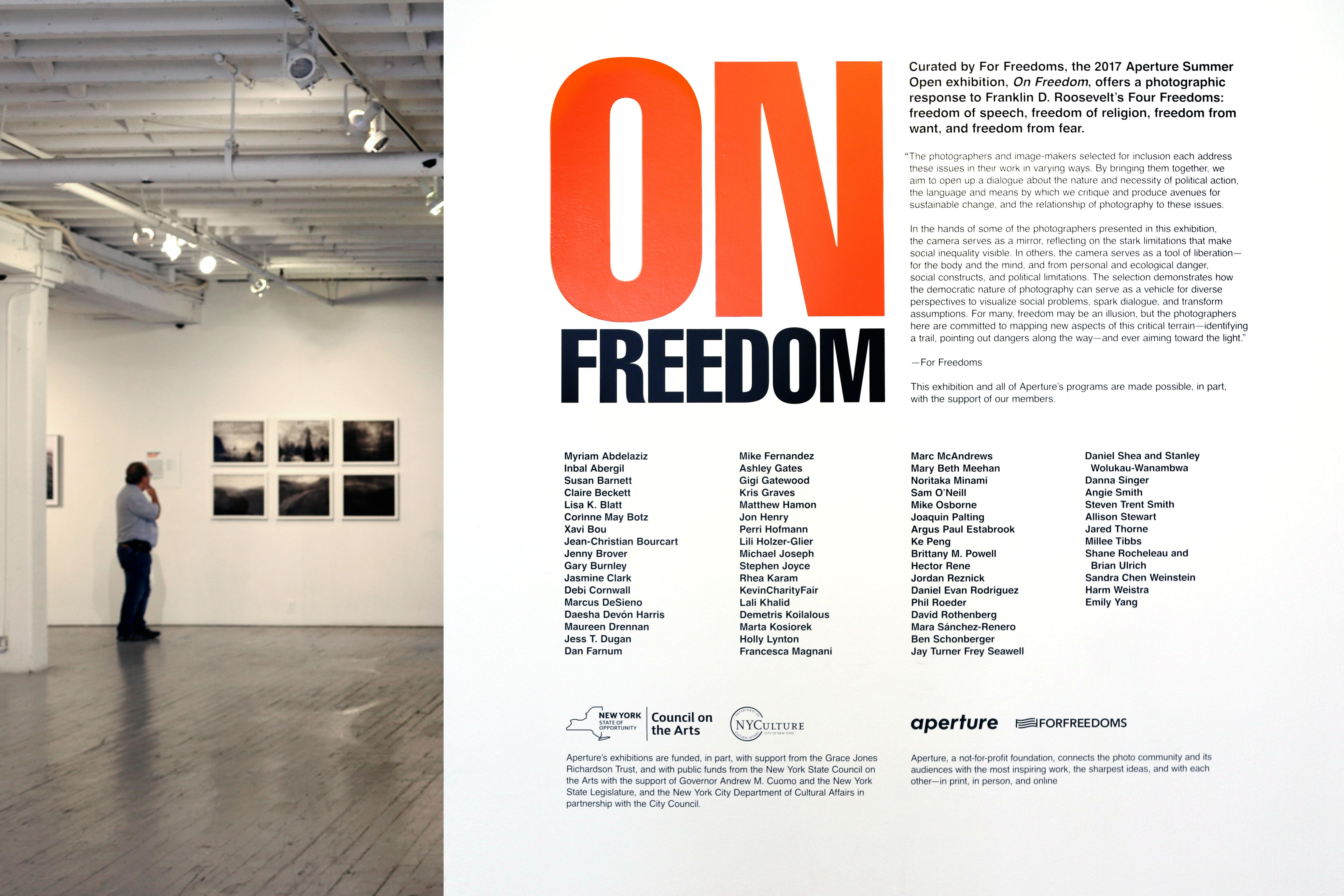The brochure or magazine article titled "On Freedom" promotes the 2017 Aperture Summer Open Exhibition curated by For Freedoms. The exhibition, inspired by Franklin D. Roosevelt’s Four Freedoms—freedom of speech, freedom of religion, freedom from want, and freedom from fear—features photographic contributions from various artists. The left side of the brochure showcases an image of an older man, dressed in black pants and a white shirt, thoughtfully observing six black-and-white photos displayed in a minimalist gallery space with white walls, a wooden floor, and ceiling lights. The only splash of color in the otherwise gray and off-white design is the bold orange-red "On" in the title, "On Freedom," with the rest of the text in black. The text-heavy right section of the brochure lists numerous contributing artists and supporting organizations, including the New York State Council on the Arts, NYC Culture, and Aperture. The overall atmosphere of the brochure is subdued, matching the serious and contemplative nature of the exhibition.